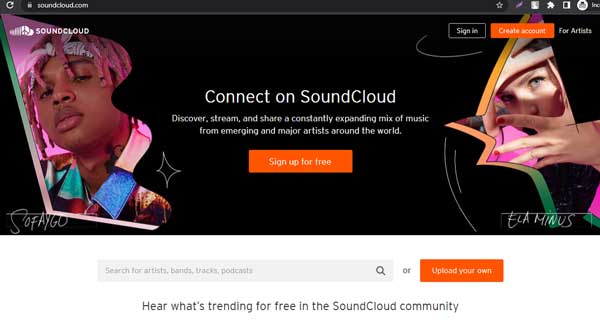The image depicts the homepage of the SoundCloud website. The URL "soundcloud.com" is visible in the top left corner. On the top right, there are several icons providing access to different options. Beneath these icons, a large black panel prominently displays images of two artists: Sofego on the left and Elaminas on the right. Their names are written in a casual, scribbled style beneath their respective images for identification.

In the center of the screen, white lettering reads "Connect on SoundCloud," accompanied by a brief description below it. An orange "Sign Up for Free" button is centrally positioned just below this text. Towards the upper right corner, there's a "Sign In" button in black with white lettering, a "Create Account" button in orange with white lettering, and a link labeled "For Artists."

At the very bottom of the screen, a search bar allows users to enter queries for artists, bands, tracks, and even podcasts. Additionally, there is an option to upload your own music, ideal for artists or music creators looking to share their work.